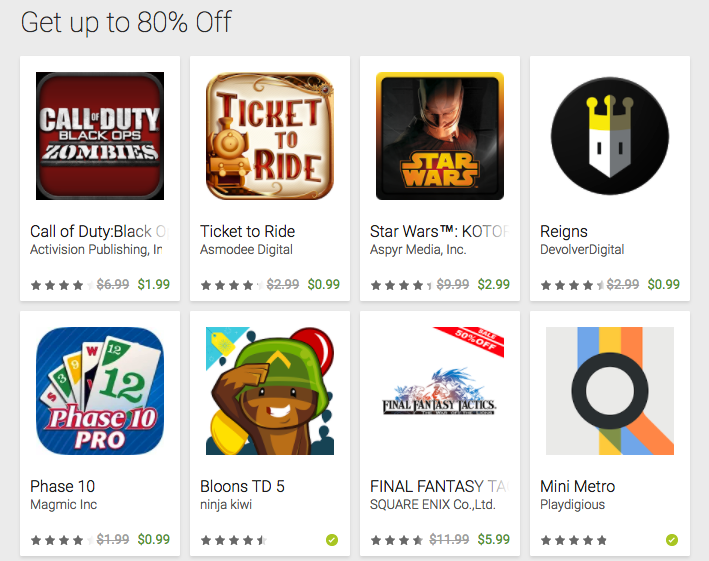This image showcases an online store for games, prominently displaying a banner in the top left corner with the text "Get up to 80% off" written in black on a grey background. Below the banner, there are eight games featured, organized in two rows with four games each.

Starting from the top left, the first game is "Call of Duty: Black Ops Zombies," which has a red background and its title in white. It is priced at $1.99, indicated in green, and has a 4-star rating.

Next to it is "Tickets to Ride" by Asmodee Digital, with a price of $0.99 and a 4-star rating.

Moving to the right, the third game is "Star Wars" developed by Aspyr Media Inc., priced at $2.99 with a 4.5-star rating.

The last game on the top row is "Reigns" by Devolver Digital, also priced at $0.99 and rated 4.5 stars.

On the bottom left, the first game is "Phase 10" by McMick Inc., which is priced at $0.99 and has a 4-star rating.

Next is "Bloons TD5" by Ninja Kiwi, with a price of $0.99 and a 4.5-star rating. This game has a green tick mark indicating it has been purchased.

Following that is "Final Fantasy" by Square Enix Co. Ltd., priced at $5.99 and rated 4 stars.

The last game on the bottom right is "Mini Metro" by Playdigious, which boasts a perfect 5-star rating and is marked as purchased, with the price displayed in dollars.